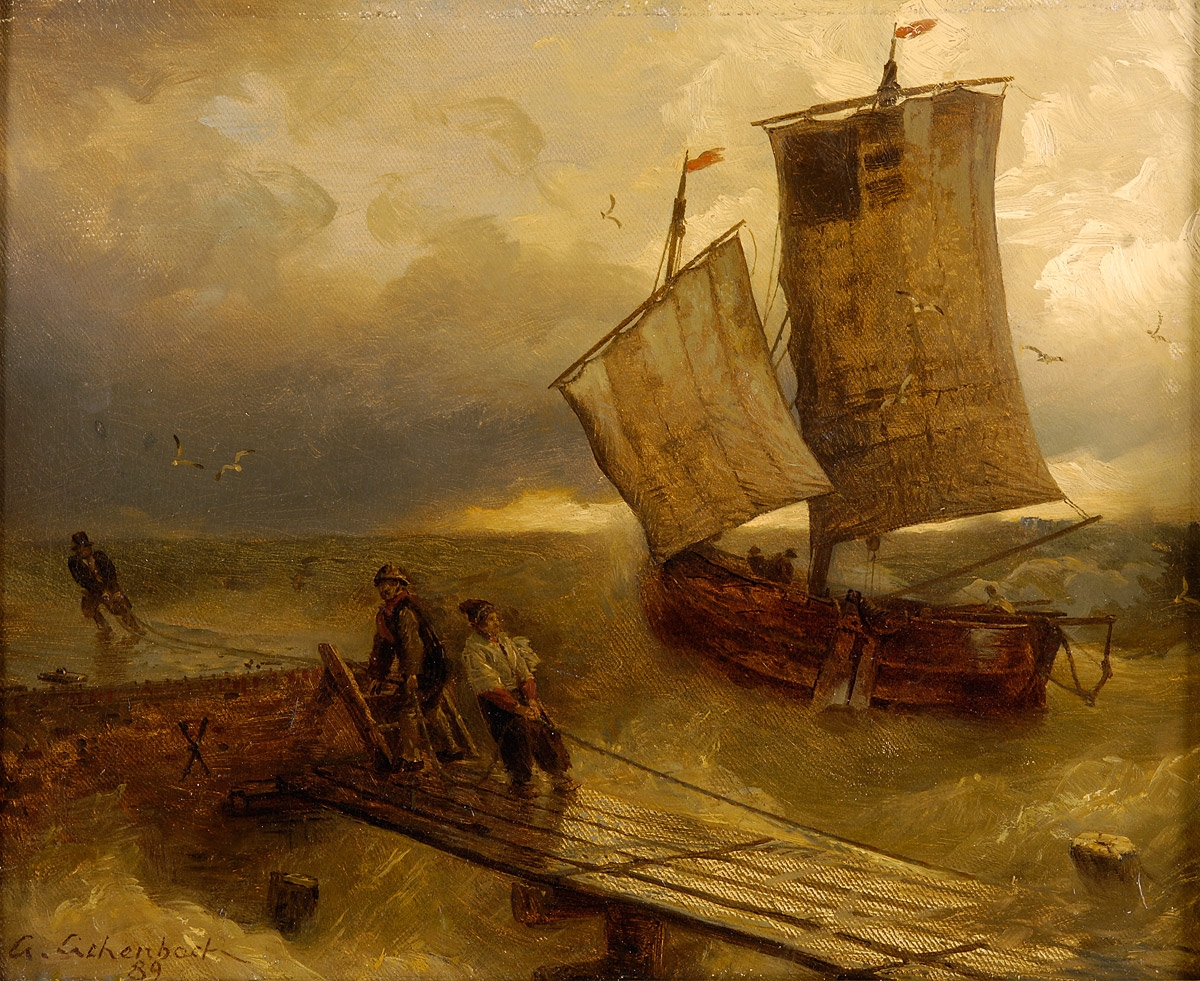This painting depicts an intense maritime scene set against a turbulent, stormy sky dominated by hues of gold, brown, and gray. In the center and to the right, a large, brown wooden ship with rectangular white sails and red flags catches the eye. The ship, reminiscent of 17th or 18th-century design, carries three figures who seem to be navigating through rough waters. The golden-toned sea is animated with crashing waves that threaten the vessel and a nearby makeshift dock or barge. On this dock structure, two individuals struggle with a rope, indicating they might be pulling something aboard or securing the vessel amidst the chaos. Seagulls fly overhead, adding to the dynamic atmosphere. The lower-left corner of the painting shows an inscription, likely denoting the artist's signature, adding a personal touch to this vivid portrayal of human endeavor against nature's might.